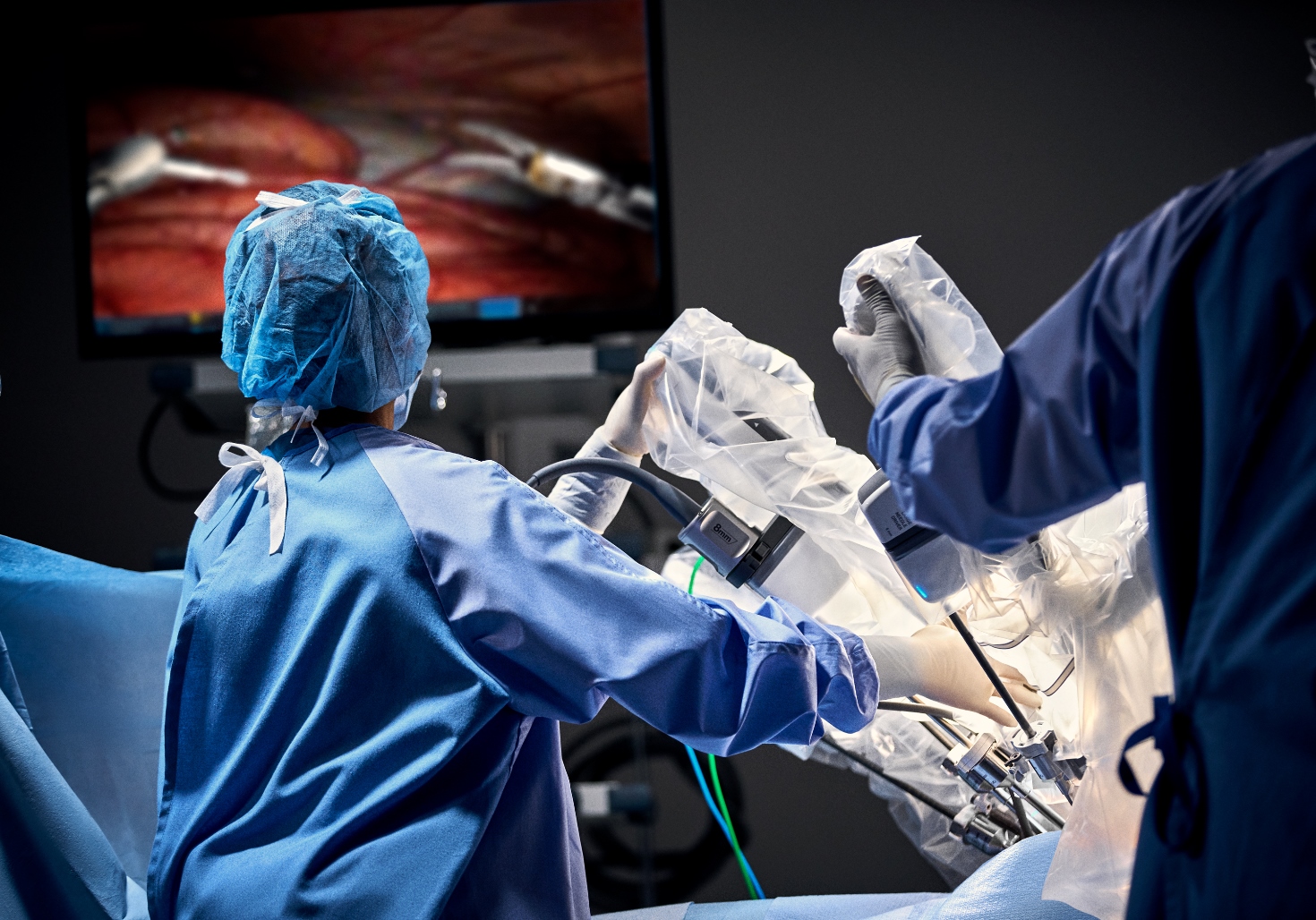This photograph captures a detailed scene inside an operating room, where two surgeons wearing blue scrubs, caps, and gloves are engaged in robotic surgery. The surgeon on the left, seen in blue scrubs and a blue-tinted cap, is positioned with their left hand holding an instrument covered in plastic and their right arm resting on a large apparatus. Visible above their right forearm is a cylindrical white piece with a black component atop it, from which a large gray cord extends upwards. In the foreground to the right, another person partially visible and also in blue or blue-green scrubs holds an instrument with their left gloved hand. Both surgeons are focused on a large black monitor mounted on a gray wall in the background, displaying real-time imagery of red and pink tissue with surgical instruments at work. The entire setup indicates a complex robotic surgery, emphasizing the precision and coordination required for such medical procedures.